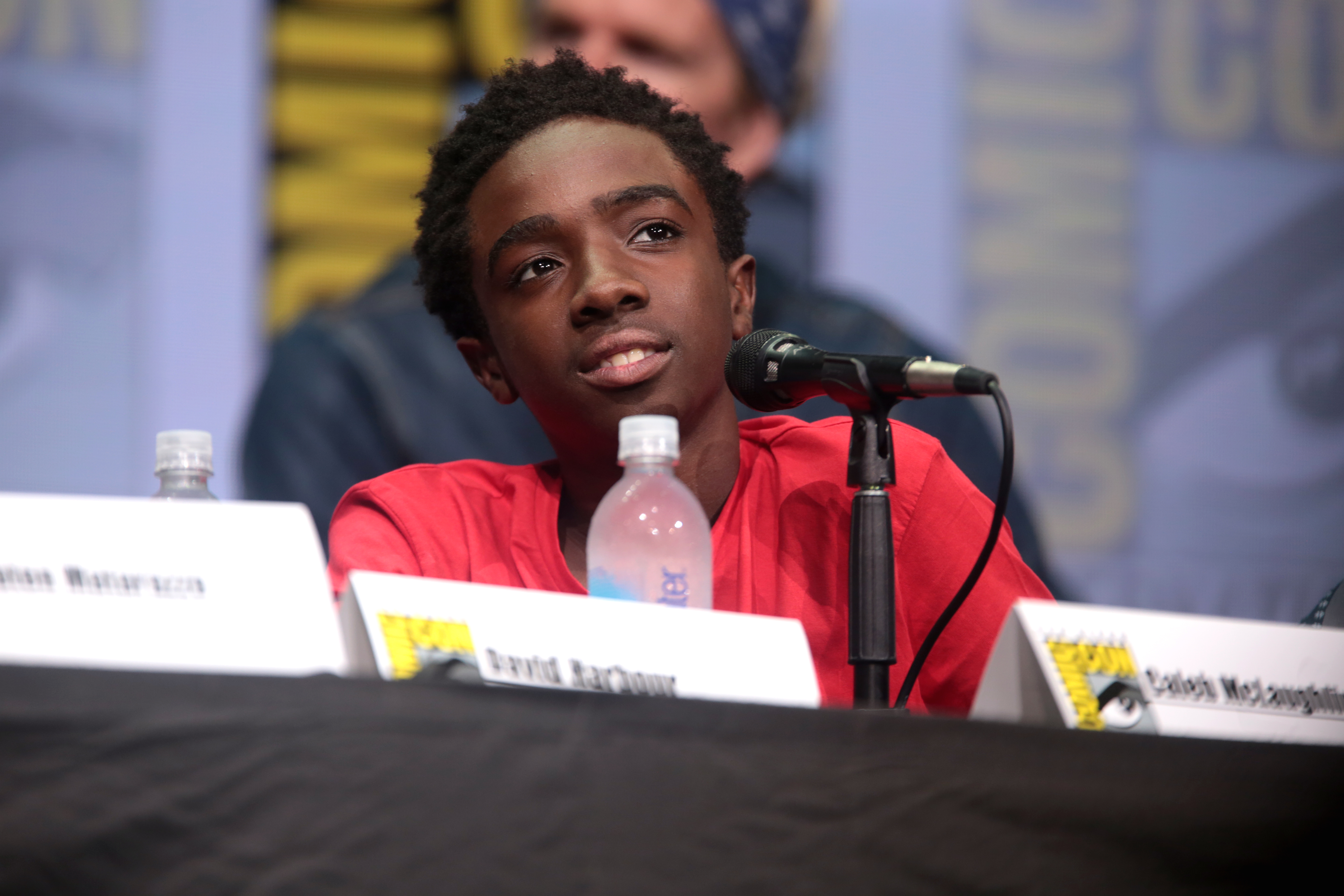The photograph showcases a young man seated behind a table covered with a black tablecloth in the foreground. The table is adorned with multiple name tags, which are folded pieces of paper featuring the Comic-Con logo and black text that is out of focus and illegible. Among the name tags, there are clear bottles of water with white caps. Positioned on the table is a black microphone stand with a microphone pointed toward the young man, connected to a black wire trailing down to the table. The young man, who is only visible from the chest up, sports a red short-sleeved t-shirt and has short black hair. His body is slightly turned to the left, and he gazes upward toward the top right of the image with his mouth slightly open, revealing his front teeth. Just behind him is an older man, partially obscured, possibly standing or sitting on an elevated platform; he appears to be wearing dark clothing and a bandana. The background features a wall adorned with multiple Comic-Con logos.